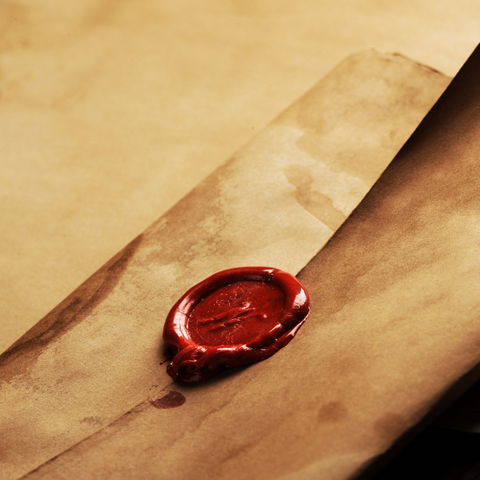The image depicts an old, weathered parchment folded into an envelope, sealed with a dark red, waxy stamp. The parchment, off-white with black and dark stains, retains a historical ambiance, possibly reminiscent of the late 1700s. The dark red wax seal, centrally placed, features a sideways uppercase "N." This intricate detail binds the envelope, indicating the formal closure. The envelope rests on similarly aged, tea-stained papers, evoking an antique setting. Darker stains appear near the seal, with a noticeable dark half-circle stain toward the bottom middle of the envelope. The background continues the theme with more aged paper, and the bottom right side of the image fades into a darker, possibly table-like surface.